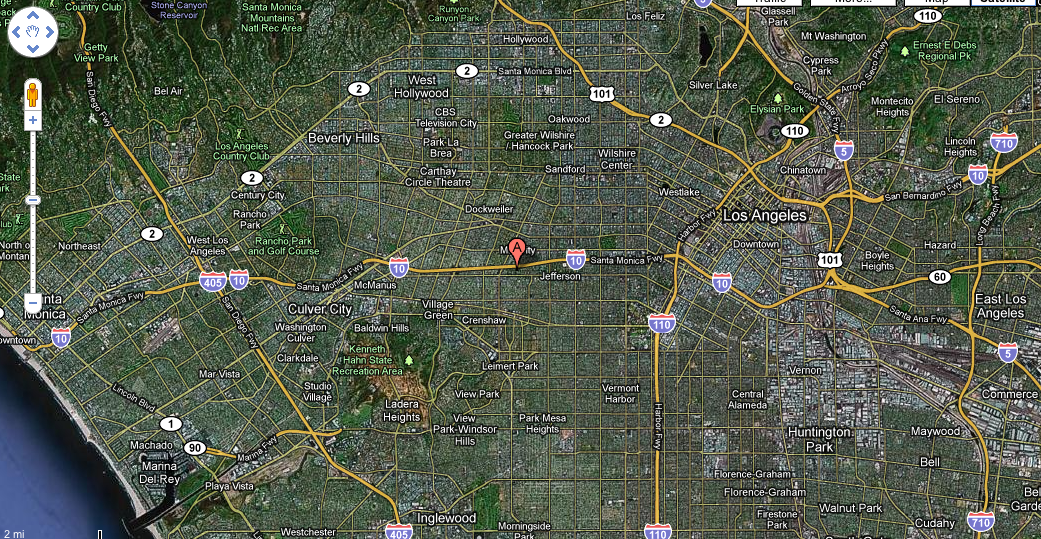This large, horizontally-oriented image depicts a hybrid GPS map combining satellite imagery with an overlay of roads and markers. The map centers on the Los Angeles, California area, showcasing a detailed view of various highways and streets. In the bottom left corner, a small patch of blue indicates the presence of the Pacific Ocean, likely southwest of Marina del Rey. The primary focus of the map is the dense urban network of Los Angeles, including major highways such as Highway 10 and Highway 110, along with numerous smaller roads.

In the upper left corner of the image, standard GPS interface elements are visible: a hand icon with directional arrows for map navigation and a zoom level indicator. On Highway 10, just west of Jefferson Boulevard and situated between Los Angeles and Culver City, a prominent red "A" marker highlights a specific location of interest. It appears this pinpoint has been selected as a focal point or destination on the map. However, the point of origin or the route to this marker remains unspecified.